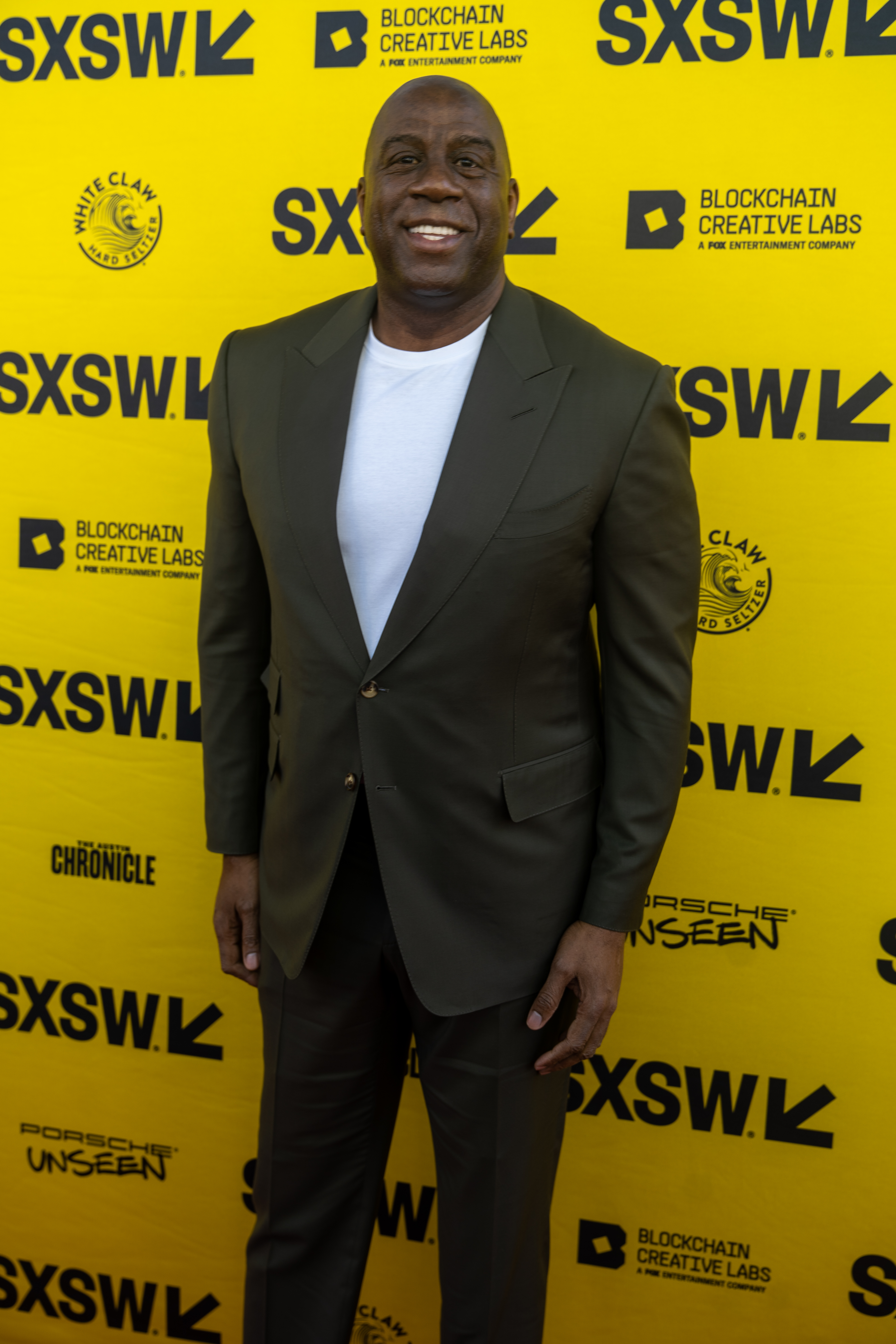This is a photograph of Magic Johnson standing in front of a yellow backdrop adorned with repeating logos and text for SXSW, Blockchain Creative Labs (a Fox Entertainment company), and White Claw Hard Seltzer. The backdrop features black text and symbols, including an arrow accompanying the SXSW logo. Magic Johnson, a tall, bald African-American man with dark eyes, is smiling broadly and looking straight at the camera, clearly posing for the photograph. He is dressed in a dark suit, which appears to be a blend of brown and black shades, paired with matching pants and a white crew-neck t-shirt underneath. His suit jacket is detailed with two buttons and what look like fake pockets on the sides. This setting suggests a red carpet or fundraising event.